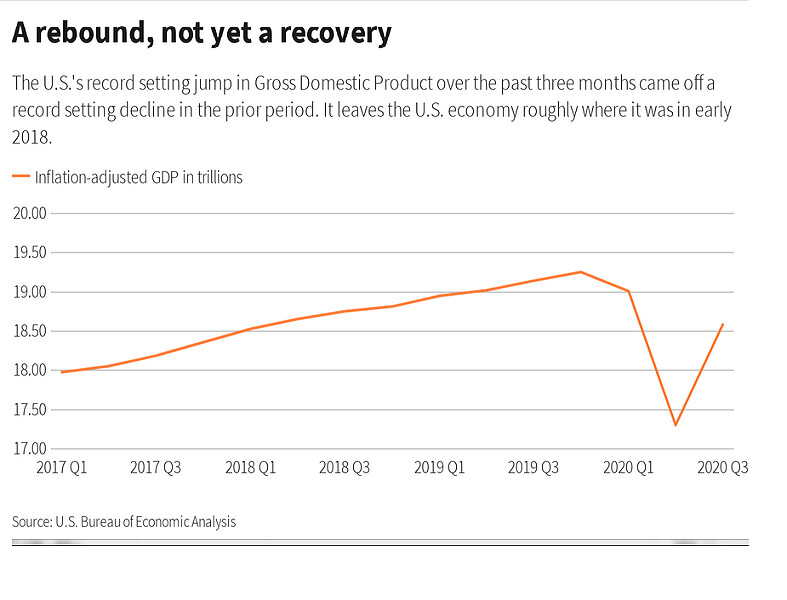This image features a detailed line graph that portrays a significant fluctuation in the U.S. Gross Domestic Product (GDP) from 2017 to 2020. The title at the top of the image reads "A Rebound, Not Yet a Recovery," and below it states, "The U.S.'s record-setting jump in gross domestic product over the past three months came off a record-setting decline in the prior period, leaving the U.S. economy roughly where it was in early 2018." The source is cited as the U.S. Bureau of Economic Analysis.

On the y-axis, the graph measures the inflation-adjusted GDP in trillions, ranging from 17.00 to 20.00 in increments of 0.5. The x-axis marks quarterly data points from Q1 2017 to Q3 2020. The graph features an orange line that begins at approximately 18.00 trillion in Q1 2017. The line shows a steady increase, maintaining an upward trajectory until Q3 2019. However, around Q2 2020, the graph depicts a sharp decline, immediately followed by an equally sharp increase through Q3 2020, indicating a volatile period. This dramatic variance highlights the unprecedented economic instability and subsequent partial recovery within the time frame.